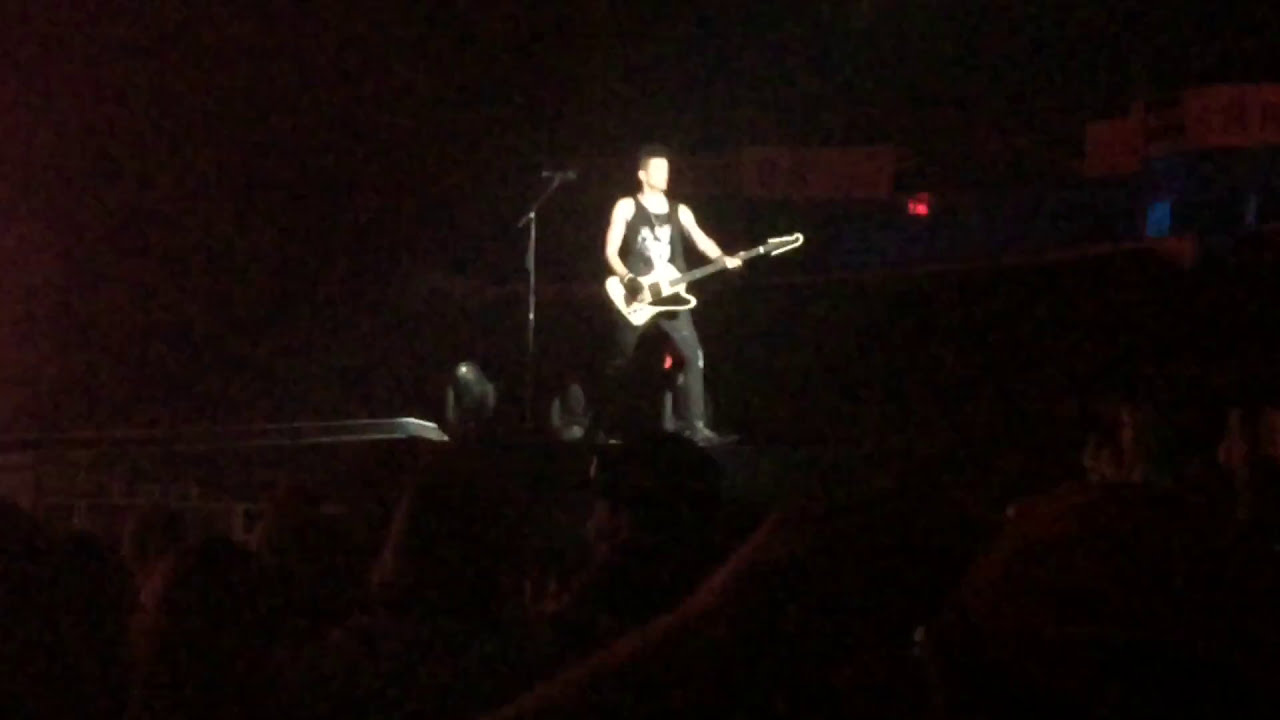This photograph captures the intense atmosphere of an outdoor rock concert from within the audience. Dominating the center stage, illuminated by bright lights, stands a musician with short black hair. He is energetically playing a white electric guitar with a black pickguard, and he is dressed in a black sleeveless shirt featuring a white design, paired with tight black pants and black boots. The musician's face is slightly obscured by the lighting, giving it a bright yellow hue, while a black microphone stand is positioned nearby, suggesting he might also be singing.

Surrounding him, the stage equipment and possibly some banners are faintly visible against the darkened background. Toward the right of the stage, a red illuminated exit sign glows. The dark contrast of the image makes it hard to discern the lower half clearly, but you can see the crowd's shadows and outlines, with several audience members raising their hands in enthusiasm. The image captures the high energy and focused intensity of the performance under dim, moody lighting.